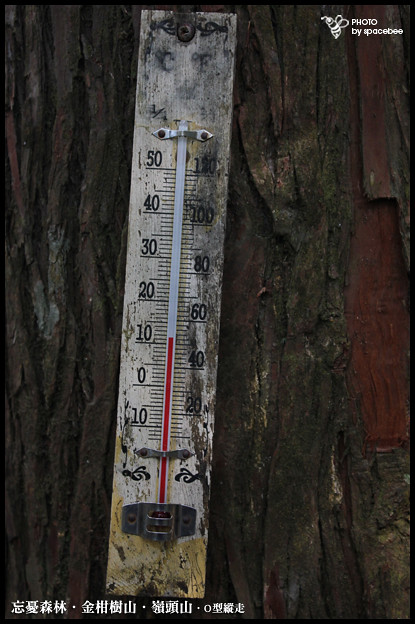Close-up Photograph of a Tree Trunk with Temperature Gauge

This detailed close-up of a tree trunk reveals its textured, thick bark with diverse lines and grains, accentuated by etchings that impart an aged appearance. The bark is predominantly reddish, with sections exposing underlayers that seem peeled back. Hints of white and yellow, resembling chalk smudges, add to the visual complexity. No leaves or branches are visible, emphasizing the trunk's intricate detail. 

In the upper right corner, there's an inscription, "Photo by Space B," accompanied by what appears to be a small bee. Affixed to the trunk is an old, tarnished temperature gauge with black smudges and grime, securely attached with a screw. It features a silver clasp at both the bottom and the top, displaying numbers along the sides. The red line on the gauge indicates a reading near 10°C and 50°F, suggesting dual scales for Celsius and Fahrenheit. At the bottom of the gauge, several white symbols point to its foreign origin.